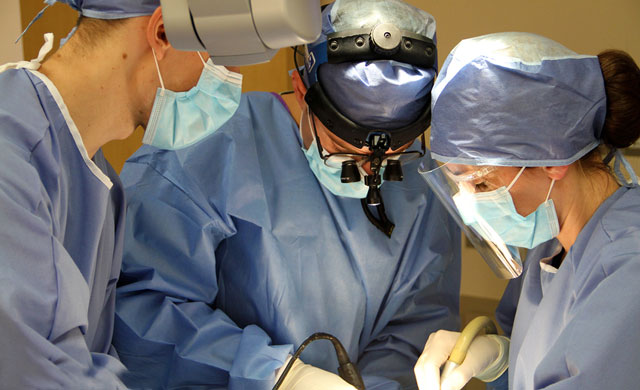The image depicts a close-up of three medical professionals standing shoulder to shoulder, focused intently on a medical procedure, evident from their head down to their waists. All three are clad in blue scrubs and protective gear: face masks, with one individual also wearing a clear face shield. The medical personnel include a Caucasian man on the left, who is faced right and dressed in blue scrubs with a face mask, a man in the center facing forward and looking down, equipped with a blue head covering, surgical glasses featuring binoculars, and holding a piece of equipment with a wire, and a woman on the right, facing left while wearing a blue head covering, mask, face shield, and white surgical gloves, grasping an instrument attached to a machinery component. The image’s detailed depiction of the scene, combined with their serious expressions and specialized tools, suggests they are actively engaged in a critical surgical procedure, reflecting a moment likely captured for educational or professional medical use.